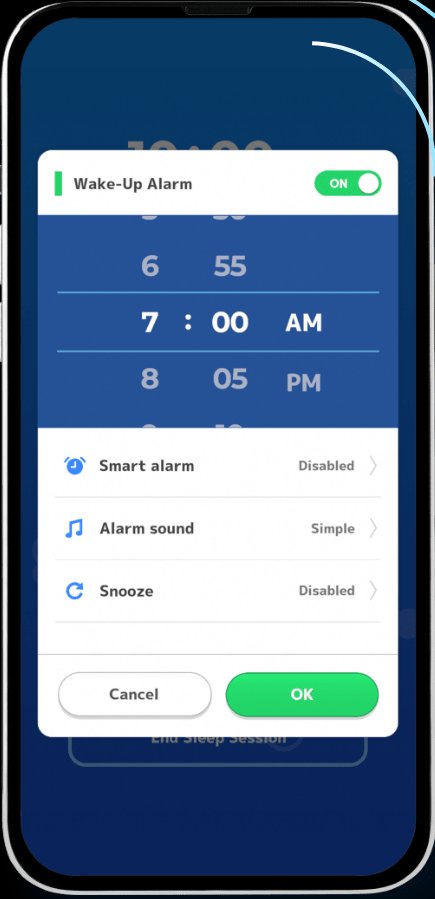This image is a screenshot of a mobile phone screen displaying the alarm settings interface. The background is predominantly blue, and there is a prominent white banner at the top labeled "Wake Up Alarm." Next to this label, there's a green upright slot and a green light beside it which indicates the on/off status of the alarm. The alarm is set for 7:00 AM, suggesting it is configured for an early morning wake-up. Below the main alarm time setting, there are additional options including "Smart Alarm: Disabled," "Alarm Sound: Simple," and "Snooze: Disabled." At the bottom, there are two buttons: "Cancel" and "OK," offering the choices to either discard or save the settings. This detailed interface hints at a customizable alarm feature, showing several slots for different settings that can be adjusted according to personal preferences.